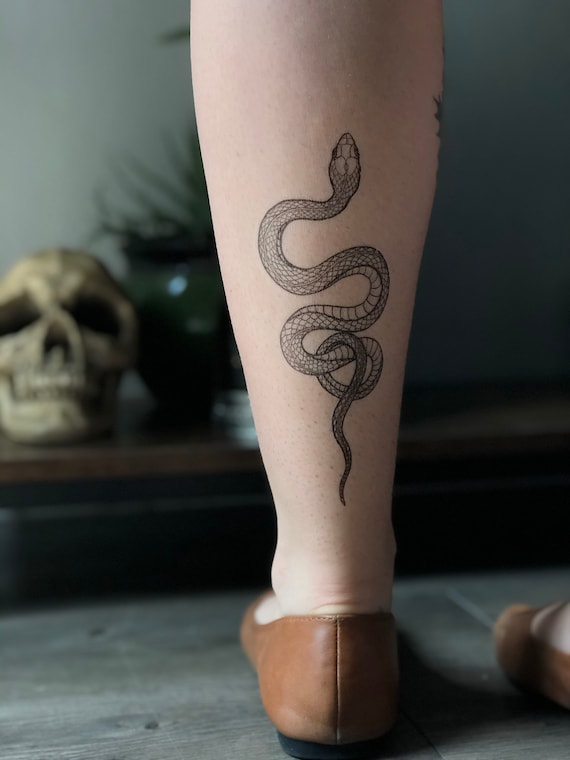This detailed photograph captures the back of a woman's left leg and calf, highlighting a striking, intricate snake tattoo in black and gray ink. The serpentine snake, designed in a diagrammatic style, elegantly swirls and knots at the bottom of her pale-skinned calf. She is adorned in brown leather flats, standing on a light gray and brown wooden surface. In the blurred background, a wooden desk can be discerned, topped with a human skull and a potted plant, adding a touch of mystique to the setting. The image also offers a glimpse of her right foot and another partially visible tattoo on the side of her left calf, enhancing the overall detailed and intriguing composition.